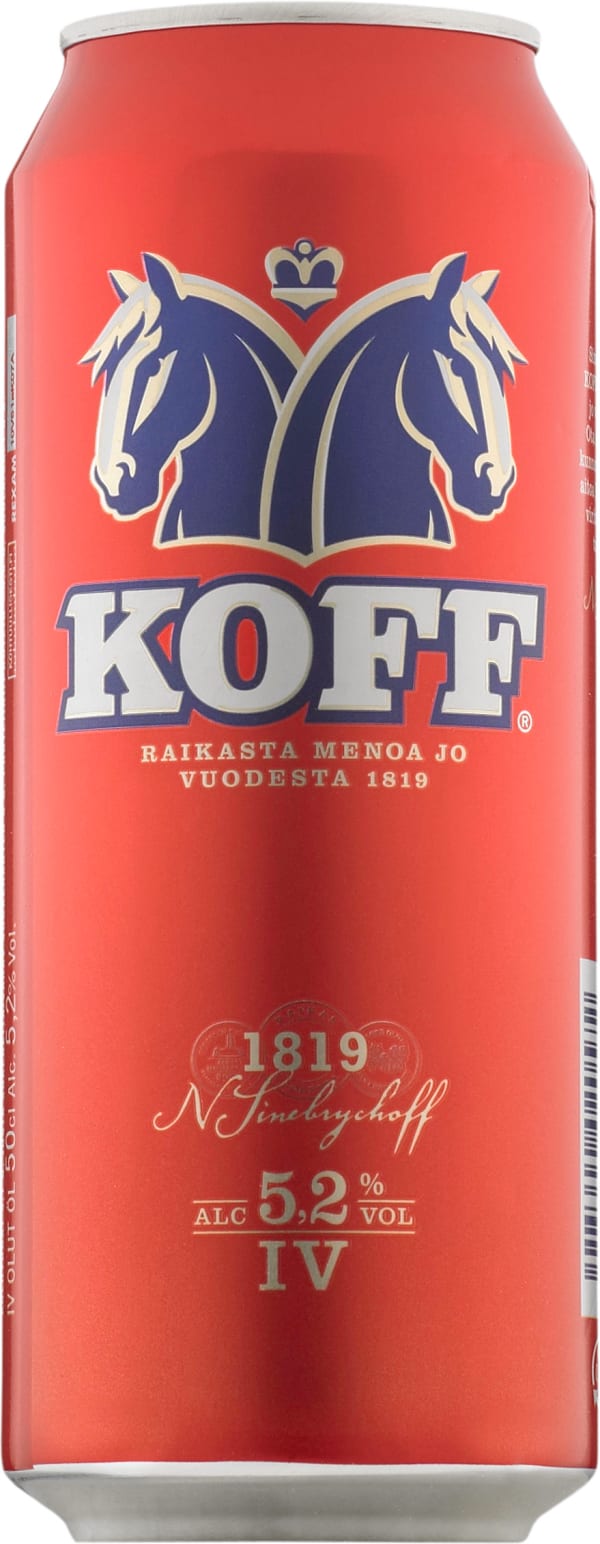This image is a detailed, color photograph in portrait orientation, featuring a tall, cylindrical can of beer named Koff, with a slight taper towards the top. The can is predominantly red with a silver bottom. Near the top center, there are two identical blue horses outlined in cream, facing opposite directions, flanking a small crown symbol of the same color scheme. The brand name "KOFF" is prominently displayed below in bold, cream-colored letters with a dark blue outline, accompanied by a registration mark. 

Underneath the brand name, there is a line of text in a foreign language: "R-A-I-K-A-S-T-A-M-E-N-O-A-J-O-V-E-O-D-E-S-T-A-1819," written in cream. This is followed by the date "1819" and a signature in the same cream color. Below that, the alcohol content is indicated as "ALC 5.2% VOL" in blue letters. On the lower right side of the can, part of a UPC barcode is visible. 

The overall style of the image is realistic and representational, capturing the product in a clean and detailed manner against a white background, suggesting a professional studio setting.